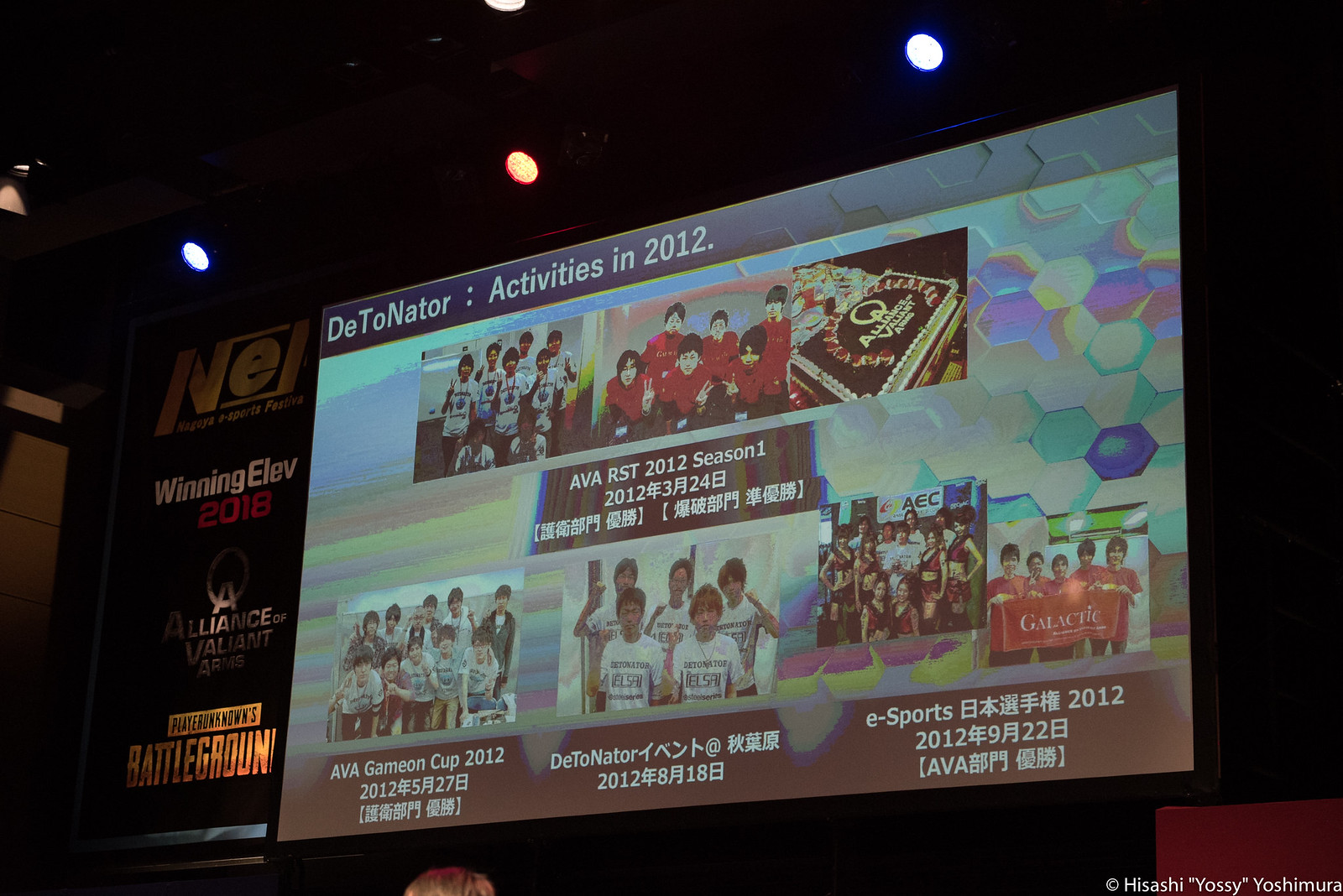The image captures a large, diagonally tilted screen on a stage, positioned centrally within an indoor setting, potentially a convention. Above the screen are three circular ceiling lights, two white and one red, illuminating the scene against a dark backdrop. The screen's upper section features a blue rectangle with the text "Detonator Activities in 2012." Below this title, on a vibrant rainbow-colored geometric background, are three images of various teams. Further down, under a text reading "ABA RST 2012 Season 1," set against a somewhat rainbow-grayish background, are four additional team pictures. The screen includes Chinese characters underneath this text, likely providing more context or information about the teams or event. The vivid color palette includes shades of black, blue, orange, purple, green, pink, yellow, brown, and gold, suggesting a lively and energetic atmosphere, indicative of an eSports or similar competitive event.